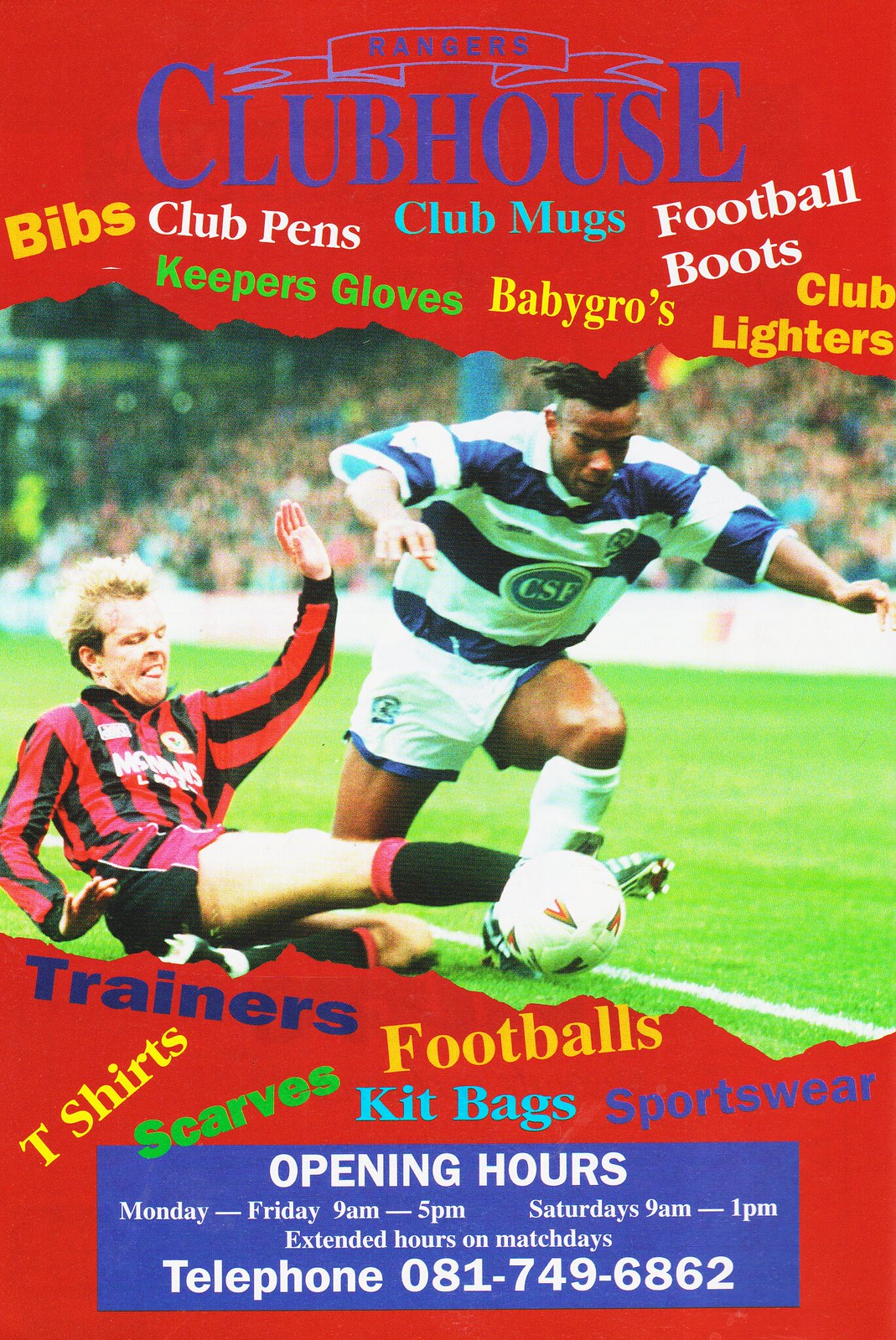The advertisement, likely from the late 90s or early 2000s due to its slightly faded appearance, serves as a magazine cover promoting a soccer club. The top and bottom sections are predominantly red, while the main body is vibrant with blue, yellow, white, and green lettering. At the very top, "Rangers Clubhouse" is prominently displayed. Below, smaller text lists clubhouse items including Bibs, Club Pens, Club Mugs, Baby Grows, Keeper Gloves, Football Boots, and Club Lighters. In the middle of the image, two soccer players are depicted mid-game. A Caucasian man, wearing a red and black vertically striped long-sleeved jersey, is lying on the ground, awkwardly positioned with his foot on a soccer ball. Over him, an African-American man with short dreadlocks, clad in blue and white horizontally striped jersey and white shorts with blue accents, is seen running, striving to gain control of the ball. At the bottom, additional items like Trainers, T-shirts, Scarves, Footballs, Kit Bags, and Sportswear are listed. The advertisement also provides clubhouse opening hours: Monday through Friday from 9 a.m. to 5 p.m., Saturdays from 9 a.m. to 1 p.m., with extended hours on match days. A telephone number, 081-749-6862, is given for further contact.